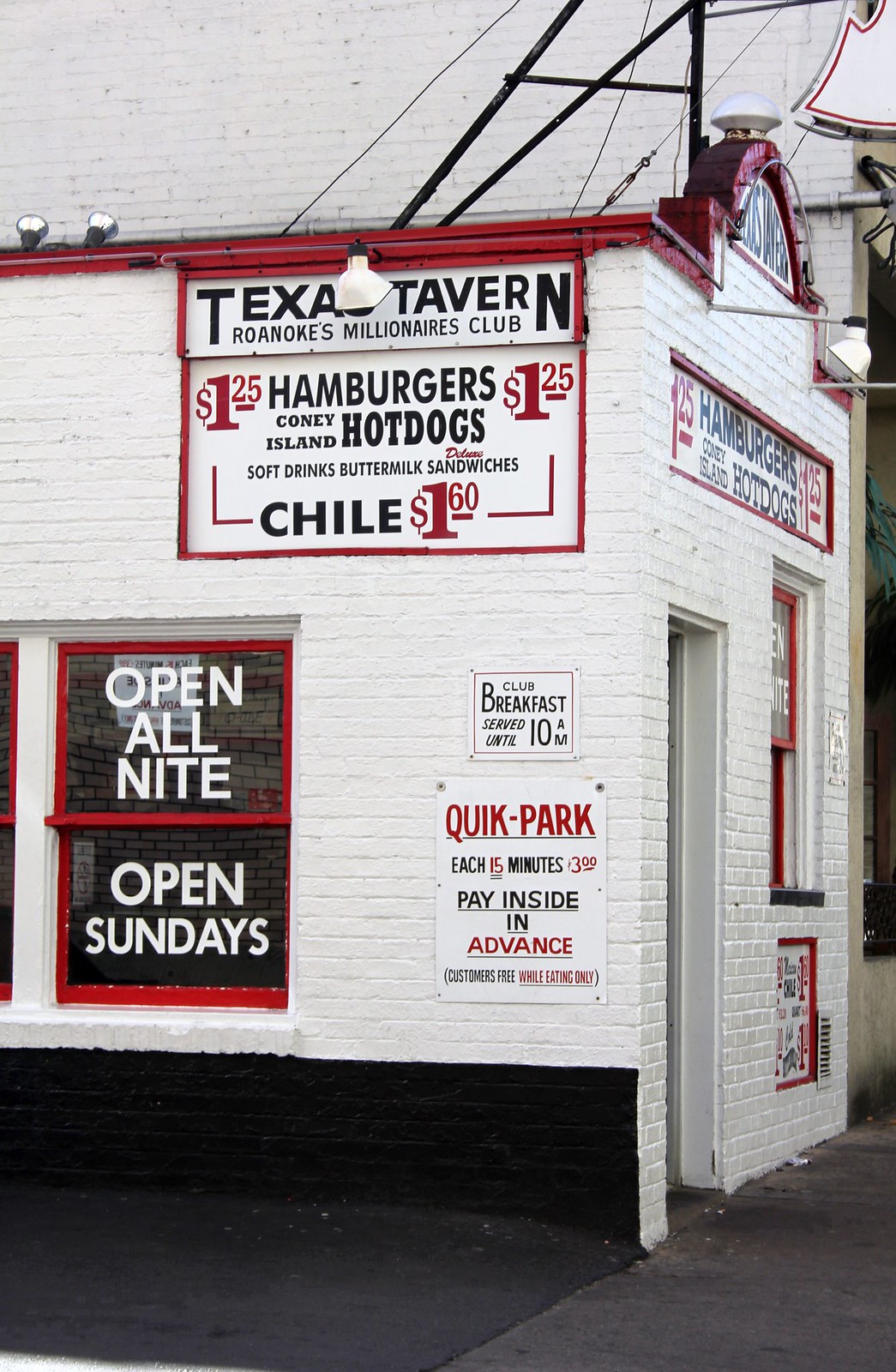This vertically oriented outdoor photograph captures a small hamburger stand, identified as Texas Tavern, situated at the corner of a white-painted brick building with its bottom layer painted black. The venue, named "Roanoke's Millionaire's Club," prominently displays a sign on its front façade listing offerings and prices: hamburgers, Coney Island hot dogs for $1.25, soft drinks, buttermilk sandwiches, and chili for $1.60. Additional signage indicates the stand is "Open All Night" and "Open Sundays," and mentions that the club breakfast is served until 10 a.m. To the right of a front door and window, there are multiple signs, including one for "Quick Park" noting each 15-minute interval costs $3.00, payable inside in advance. The building front stretches towards the right while the side wall extends to the left, bordered by a cement sidewalk. A larger sign atop the building emphasizes the establishment's name and services, underscoring its inviting, retro ambiance.